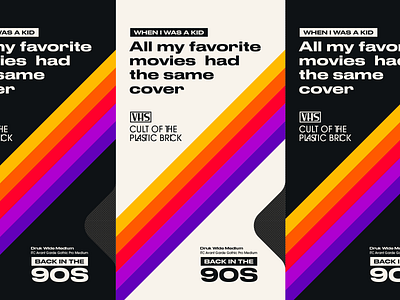The image depicts an advertisement-style design featuring three VHS cassette cover designs from the 90s arranged horizontally. The central cover is white with black text reading, "When I was a kid, all my favorite movies had the same cover - Cult of the Plastic Brick - VHS." The covers on the left and right are reversed, displaying this text in white against a black background. All three covers feature a diagonal rainbow stripe pattern that starts from the bottom left and progresses upwards towards the right in the colors of yellow, orange, red, light purple, and dark purple. The repeated text and striped motif give a nostalgic nod to vintage VHS aesthetics.